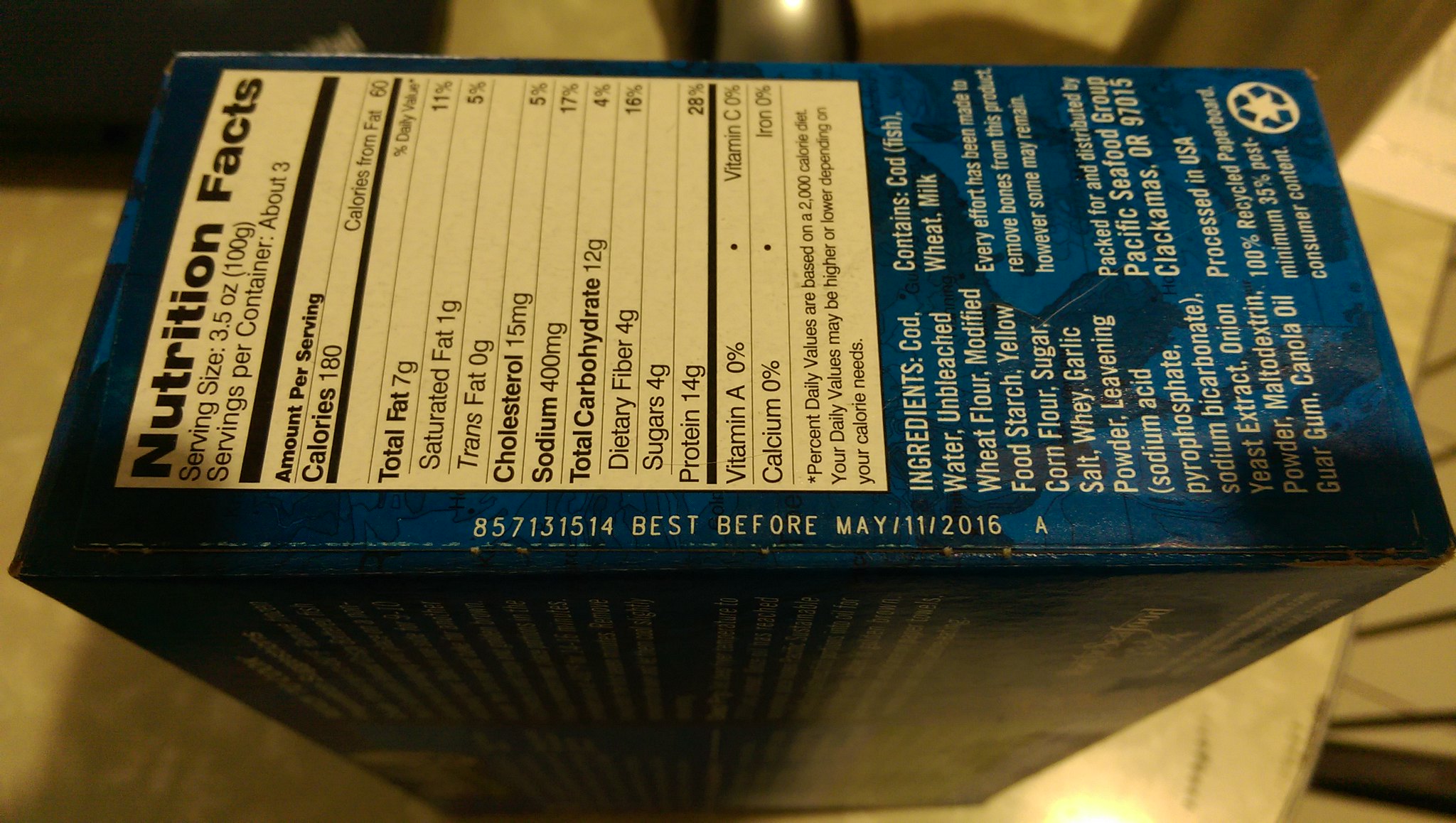The image displays the side of a rectangular blue box, reminiscent of a cereal box, containing food, specifically frozen cod fish. The box is a mix of medium and dark blue, resting on a counter. Prominently featured are the nutrition facts printed in black on a white rectangular background. Details include a serving size of 3.5 oz (100 grams), with about 3 servings per container. Nutritional information lists 180 calories per serving, 7g total fat, 1g saturated fat, 0g trans fat, 15mg cholesterol, 400mg sodium, 12g total carbohydrates, 4g dietary fiber, 4g sugars, and 14g protein. Notably, it has 0% Vitamin A and 0% calcium. The packaging also notes a 'Best Before' date of May 11, 2016.

An ingredients list reveals the contents: cod, water, unbleached wheat flour, modified food starch, yellow corn flour, sugar, salt, whey, garlic powder, leavening (sodium acid pyrophosphate, sodium bicarbonate), yeast extract, onion powder, maltodextrin, guar gum, and canola oil. The box includes warnings that it contains cod (fish), wheat, and milk. There are no images of the actual product visible in the photo, affirming that it is indeed a box of frozen cod fish.